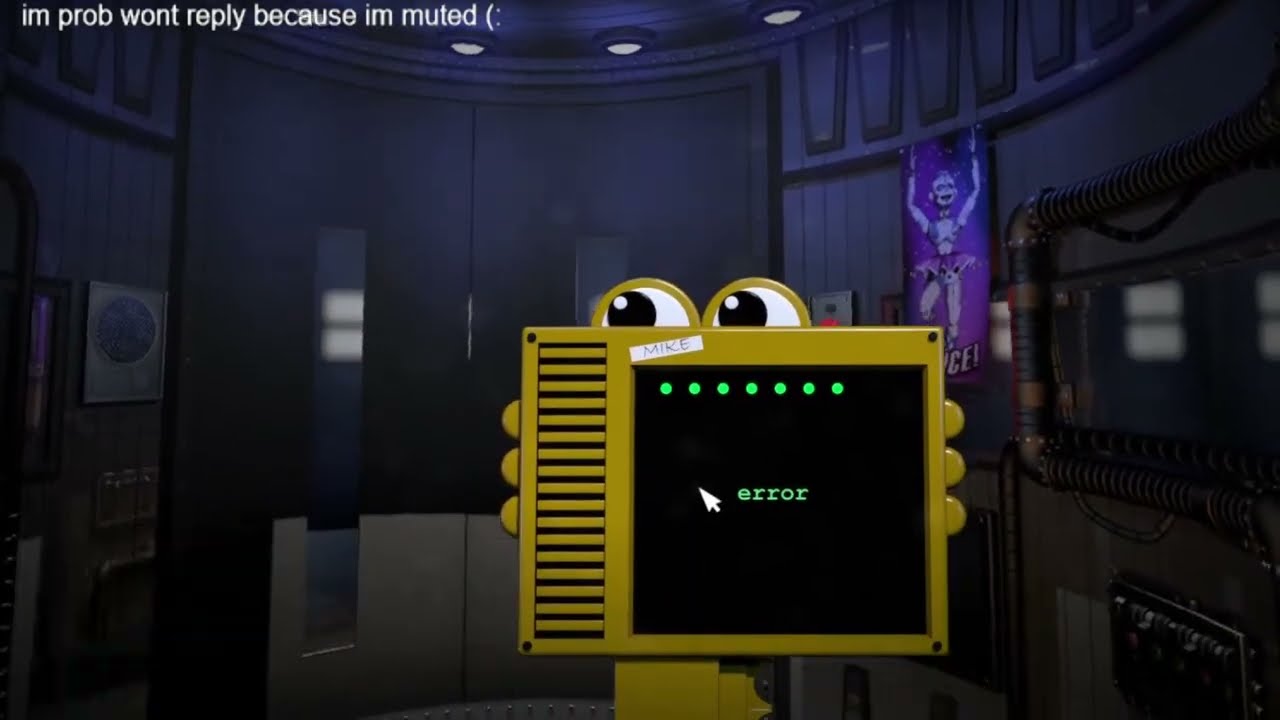The image depicts a scene from a video game, likely from the "Five Nights at Freddy's" series. At the center of the image, there is a cartoon-like yellow machine with two eyes on top, gazing to the right. This machine sports three bumps on each side resembling fingers holding a screen. The screen is black with green text that says "error" in the middle, accompanied by a collection of dots at the top. Above the machine, the interface displays white text stating "I probably won't reply because I'm muted :)" on a dark purple background. The setting appears to be a dimly lit, rounded metallic tech room, possibly resembling an elevator, with grey metallic walls, circular and horizontal lights, and various mechanical objects including pipes and speakerphones. A poster featuring a dancing ballerina is visible on the left side of the image, adding more context to the game's eerie environment.